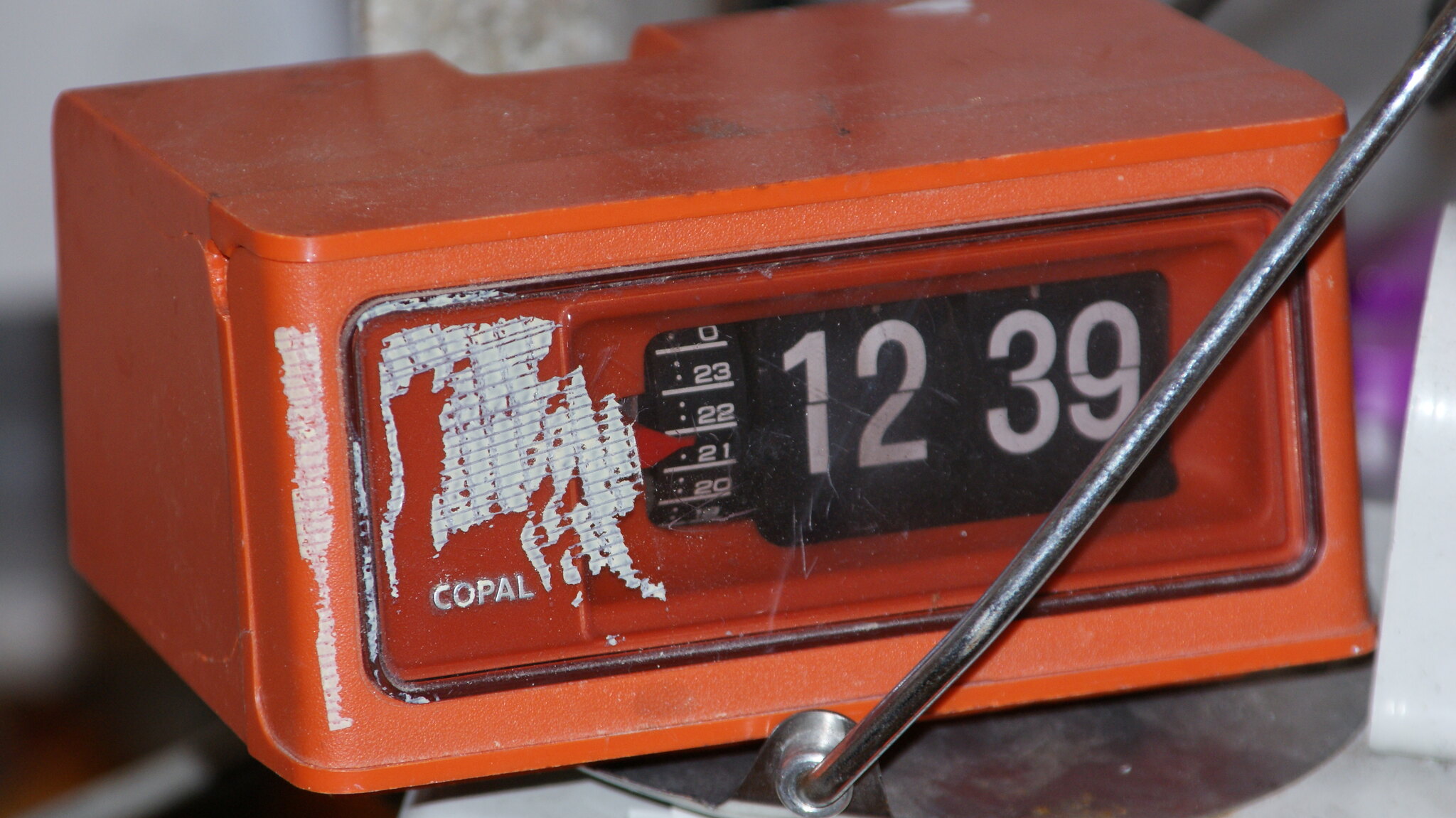This color photograph captures a close-up view of an old-fashioned alarm clock, likely from the 1970s or 1980s. The rectangular clock features an orange plastic exterior, with a flat orange top and visible surface scratches, particularly white ones on the left-hand side and the clear front cover. The clock displays the brand name "COPAL" in white text to the left. The current time shown is 12:39, depicted in large black flip-down numbers against a dark background. Additionally, there is a rotating dial nearby, set to the number 22, surrounded by other numbers such as 0, 23, 21, and 20, each separated by lines. A single stainless steel bar, presumed to be an antenna, extends upwards from the front corner of the clock.